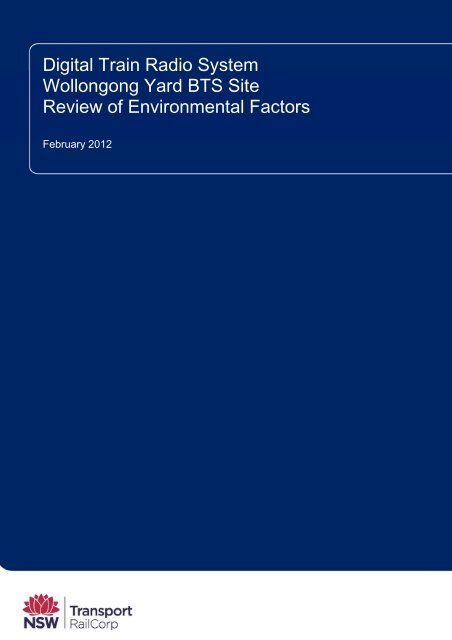The image appears to be the cover of a booklet, designed in a rich royal blue color. Dominating the top portion of the design is a prominent rectangle with rounded top and bottom left corners; it extends from the right edge almost to the left, featuring a delicate white border on three sides (top, left, and bottom). Inside this rectangle, bold white text reads: "Digital Train Radio System," followed by "Wollongong Yard BTS Site" and "Review of Environmental Factors." In smaller white text at the bottom left of this rectangle, the date "February 2012" is displayed. The bottom section of the cover features a white strip running horizontally, housing a small red flower logo with the text "NSW" beneath it. Adjacent to this logo, to the right, the black text states "Transport Rail Corp." The overall design is clean and simple, emphasizing the text and providing clear, necessary information.